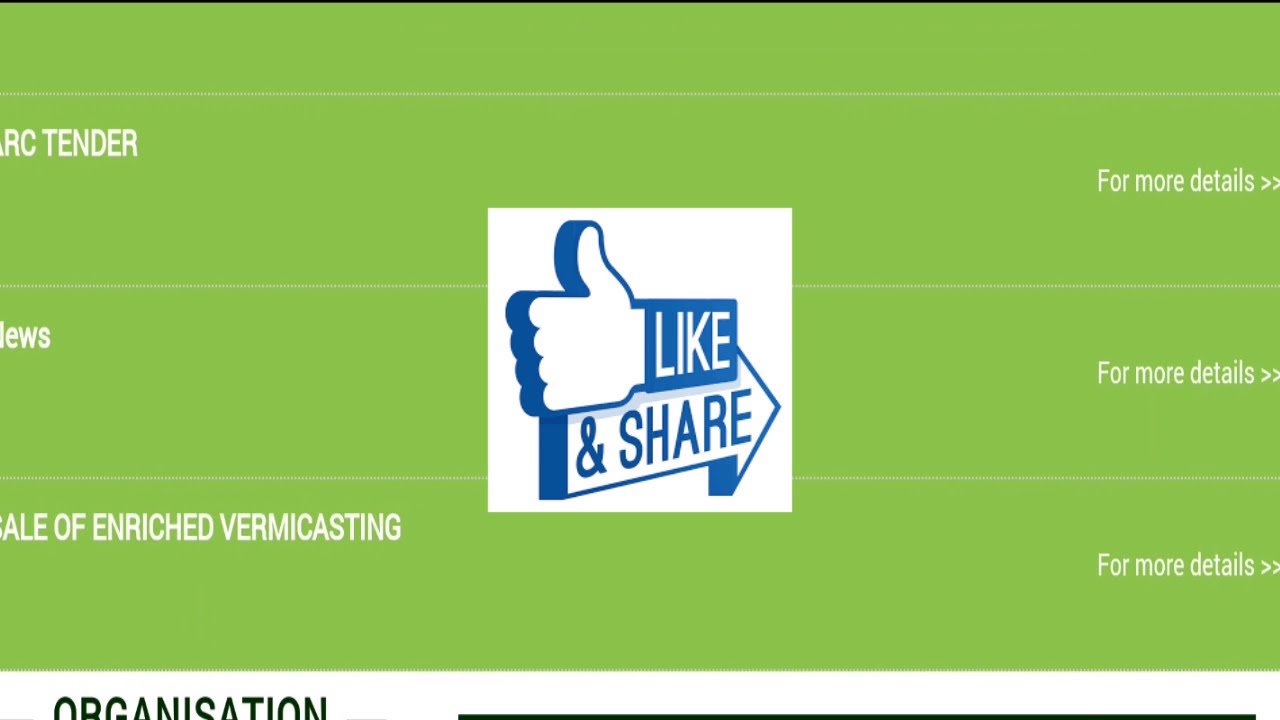The image appears to be a detailed section of a web page, featuring a medium green background with three off-white horizontal stripes separating different sections. On the left side, there is partially cropped text including "RC tender" and "sale of enriched vermicasting." The word "organization" is visible in black text on a white tab at the bottom, with a black horizontal rule beneath it. On the right side, each section displays "for more details" accompanied by two right-facing arrows. Centrally located is a white square with a 3D-like thumbs-up icon; the word "like" is written in blue above the thumb, while "and share" is written beneath it with an arrow pointing to the right. This image, possibly a screen grab from a video, resembles an end screen commonly seen on platforms like YouTube.